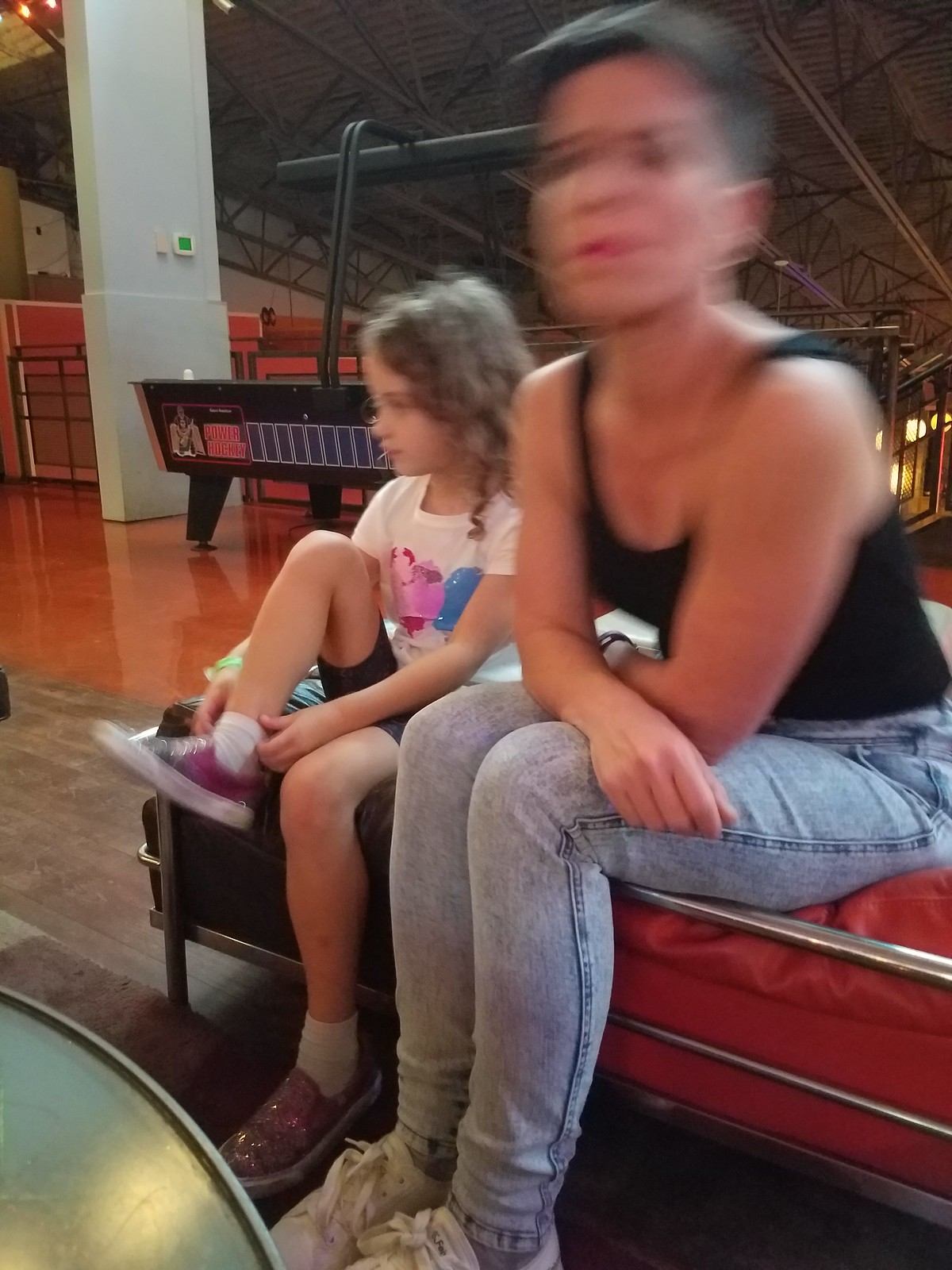In this color photograph, we see a young woman and a young girl seated on a long red cushioned bench with a chrome frame. The young woman's face is blurred, revealing minimal details except her short black hair, a sleeveless black top, blue jeans, and white lace-up shoes. She sits with her arms crossed over her knees, positioned slightly to the right in the image. The young girl, approximately six to nine years old, has brown curly hair that falls to her shoulders and is captured in profile. She is wearing a white t-shirt with a blue and pink design, black shorts, white socks, and pink and blue shoes, with her right leg lifted as if tying her shoelaces. Both are looking towards the left side of the photograph.

The bench they are sitting on runs diagonally from the lower right to the center of the image and has a horizontal grey metal bar rimmed along its top, middle, and bottom. The background suggests a gymnasium setting, featuring a grey and red floored area, a wooden industrial roof, and more benches and gym mats. In the upper left corner, there is a grey rectangular column extending from the floor out of frame. Part of a green, circular coffee table can be seen in the lower right corner, illuminated by some light reflecting off its surface. There are no text or print visible in the image.